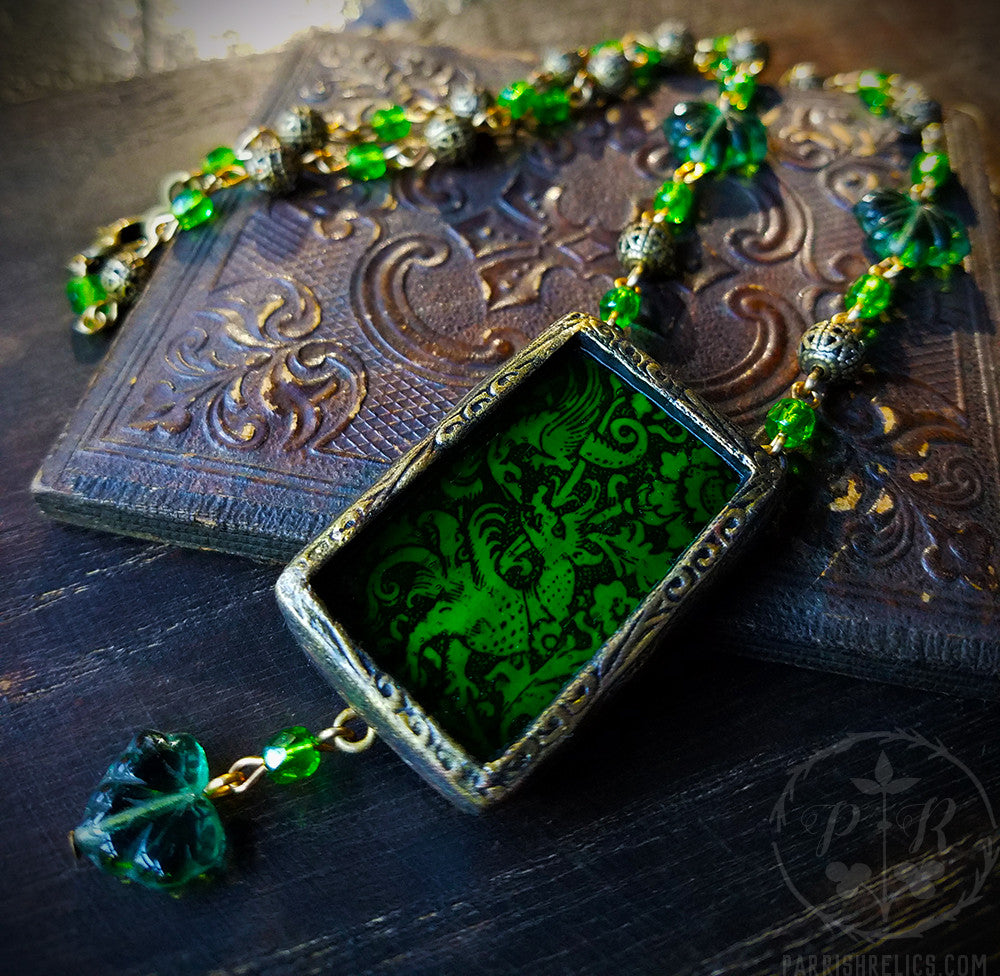A captivating necklace, seemingly with medieval flair, lies against an antiqued backdrop featuring a distinct square bronze plate adorned with potentially French or Spanish fleur-de-lis motifs. The handcrafted necklace comprises an array of intricate jade stones, designed in various forms from cylinders to spheres, leaves, and hearts, interspersed with silver embellishment balls. Its centerpiece is a striking rectangular jade pendant encased in a weathered gold or bronze frame, showcasing a carved figure that resembles a semi-human animal, potentially a fox dragon. From this pendant dangles a delicate heart-shaped jade piece, adding to the necklace's intricate beauty. The dark background, possibly a wooden surface, provides a fitting contrast that enhances the aged elegance of the piece. In the lower left corner, there's a faint inscription: "PR" encircled, followed by the text "perishrelics.com", attesting to its intriguing historical provenance.